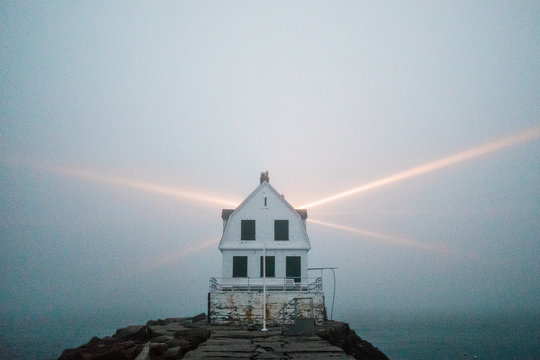The image depicts a decaying, two-story white house precariously perched on a narrow, rocky hill or cliff, set against a large, fog-enshrouded body of water. The sky is a muted gray with subtle bluish hues due to the dense fog, which veils most of the background. Despite the overcast atmosphere, rays of pinkish-orange light emanate symmetrically from behind the house, forming an X-shaped pattern, with two extending upwards at a gentle angle and two shorter beams pointing downwards.

The house, which resembles a non-traditional lighthouse, features darkened, possibly boarded-up windows—two on the upper floor and three on the lower level. The rocky base of the hill is composed of brown, slab-like stones, which appear almost black under the dim light. A flagpole stands in front of the house, devoid of any flag. Additionally, a precarious bridge or path, made mainly of stones, appears to lead up to the dwelling, adding to the eerie, isolated ambiance of the scene.